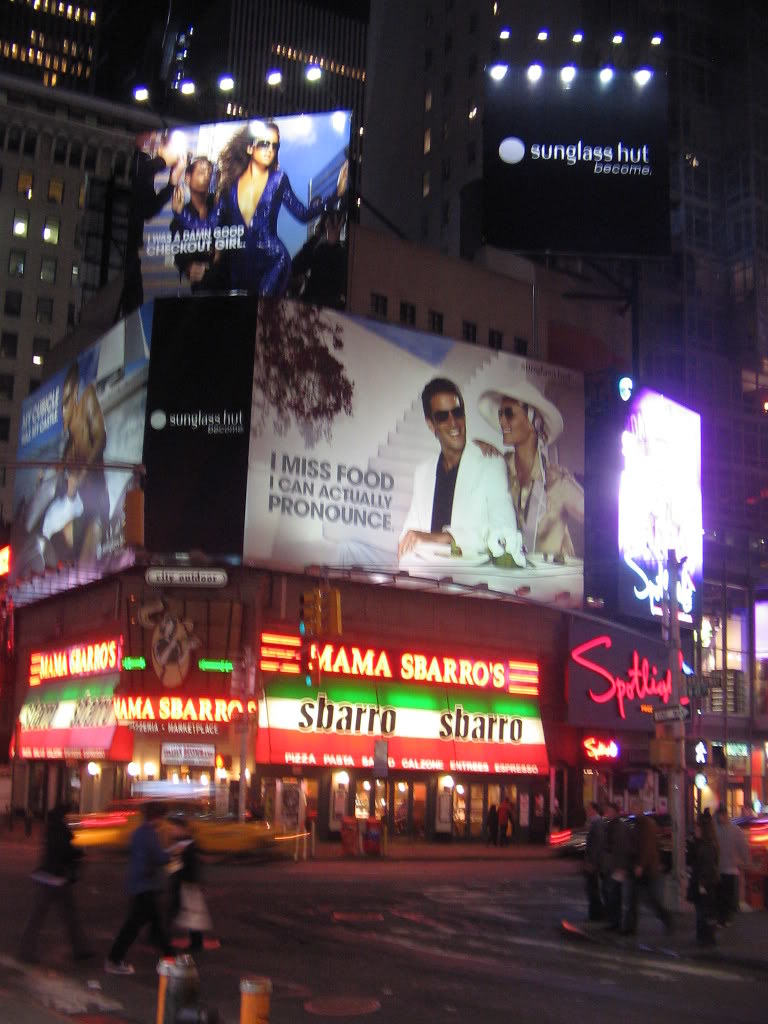A bustling urban scene showcasing vibrant LED billboards adorned above a corner-store restaurant named Mama Sparro’s. The establishment, located at the intersection of two busy streets, boasts its own array of bright LED signage on its façade. The image captures the restaurant from across the street, offering a clear view of pedestrians meandering along the sidewalks. Towering city buildings loom in the background, contributing to the lively atmosphere of the cityscape. The convergence of modern advertising and daily life epitomizes the dynamic essence of this metropolitan area.